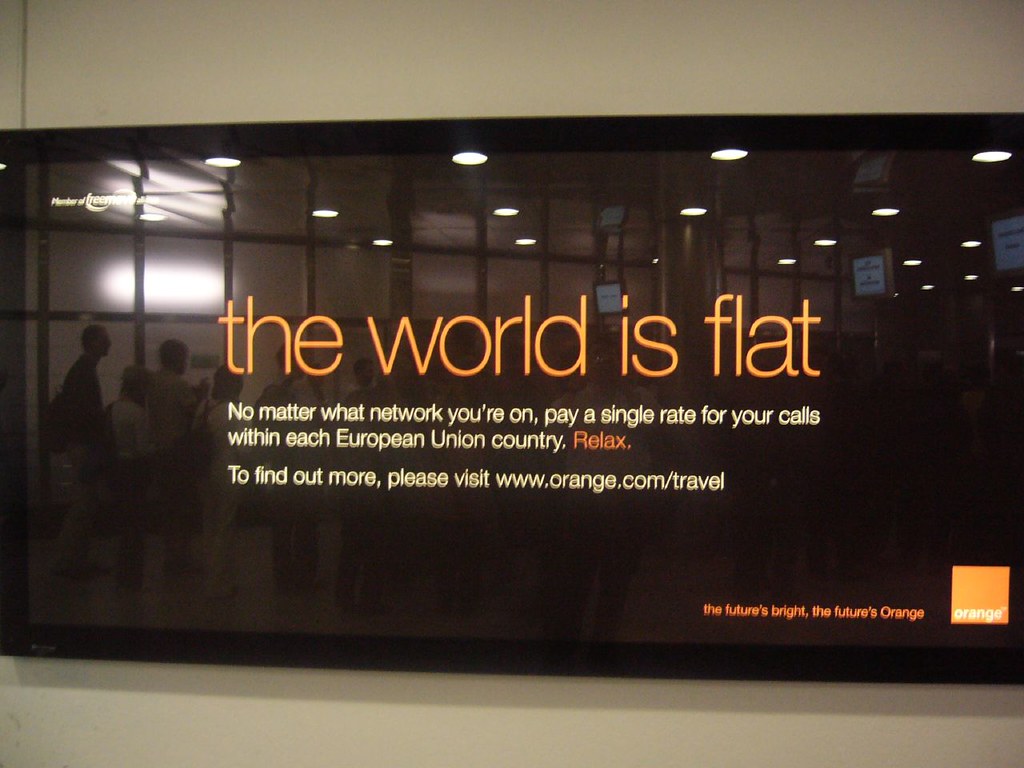In the image, a large flat-screen TV is centrally mounted on a light greenish to off-white wall, which spans the entire width of the photograph. The TV is bordered in black and features a black screen with prominent text displayed in the center. The headline on the screen reads "The world is flat" in big, bold, yellow font. Below this, there is additional text stating, "No matter what network you're on, pay a single rate for your calls within each European Union country. Relax. To find out more, go to orange.com/travel." In the bottom right corner of the TV screen, the message "The future is bright, the future is orange" is visible, accompanied by a logo—a white "orange" text inside an orange box. Reflections on the screen reveal the presence of people, lights, glass windows, and other display screens on the opposite side of the room, suggesting the setting is likely indoors at a conference. The overall color palette includes tan, off-white, black, white, orange, and gray tones.